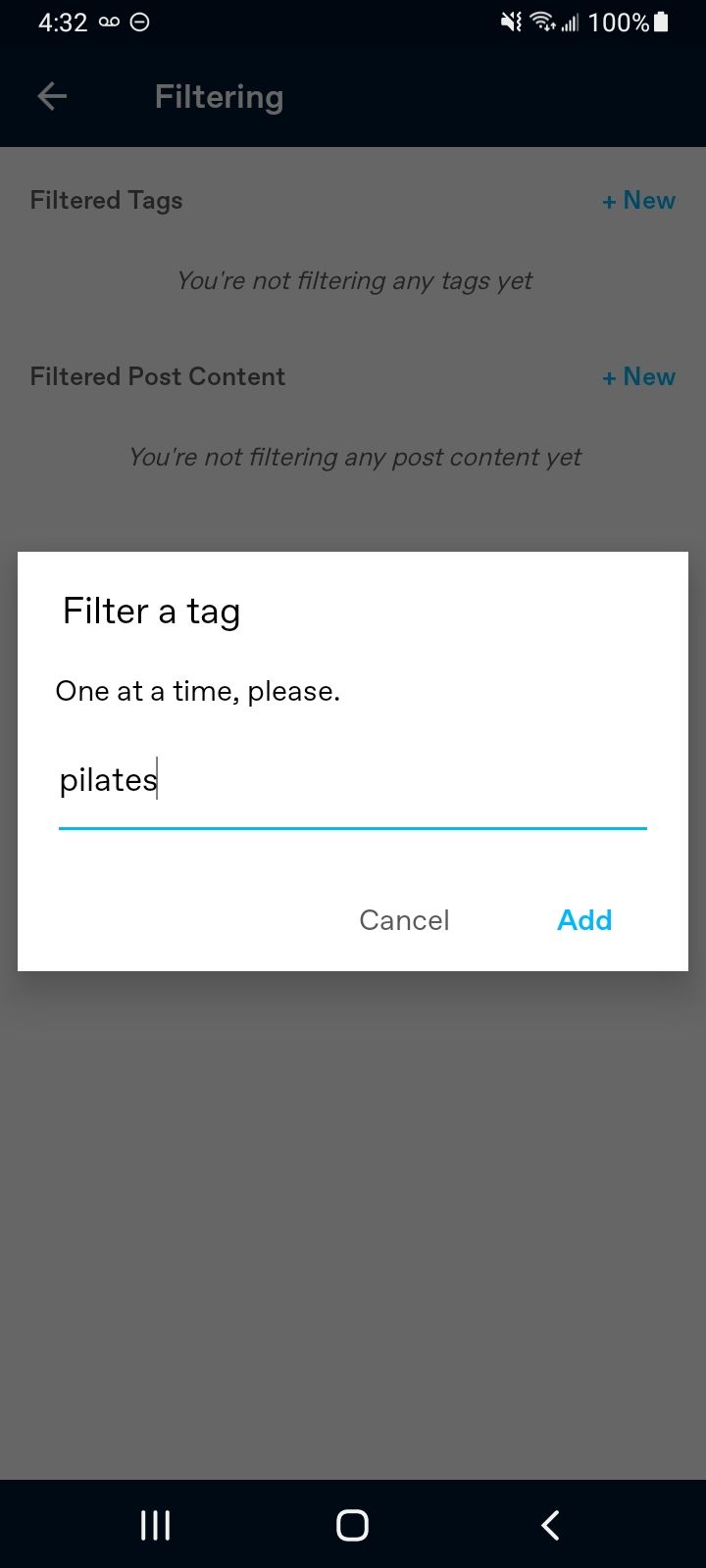The image depicts a cell phone screen with a black strip across the top. On the left side of the strip, it displays the time as "4:32". The phone is set to vibrate mode, indicated by a circle with a line through it. Additional icons show full Wi-Fi signal strength, phone signal bars, and a battery at 100%.

Below the black strip is a section showing a left arrow with the text "Filtering." The entire screen has a gray overlay, indicating a pop-up is active. The pop-up message says, "Filtered Tags: You're not filtering any tags yet. Filtered Post Content: You're not filtering any post content yet." It prompts the user to "Filter a tag one at a time please." There is a blue bar labeled "Pilates" (spelled out as P-I-L-A-T-E-S), which serves as a data field.

At the bottom of the pop-up are two buttons: "Cancel" in gray and "Add" in blue, suggesting an action to add a tag filter. The navigation bar at the very bottom of the screen displays three vertical dots, a circle, and a left arrow, standard for most smartphones. The predominant colors on the screen are white, gray, black, and blue. The gray overlay covers most of the screen, indicating that the pop-up is the active focus.